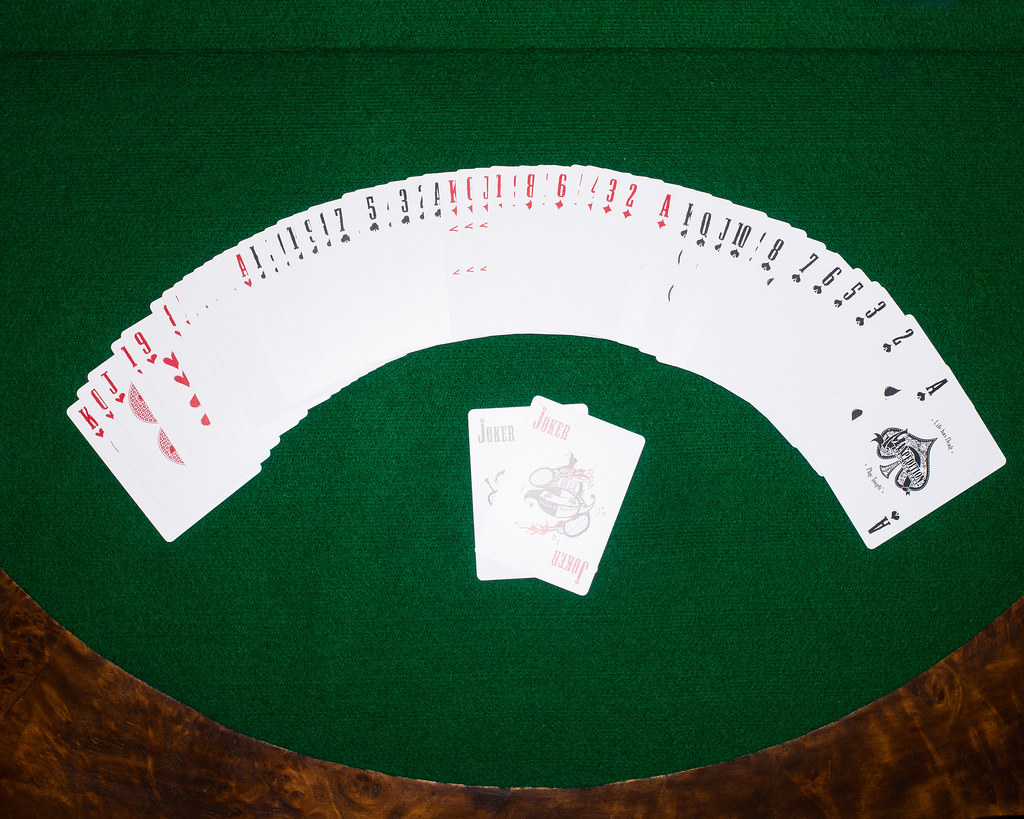A neatly arranged fan of playing cards adorns a circular poker or blackjack table, showcased against a rich green felt background typical of such tables. The table's periphery is accentuated by a patterned border featuring alternating light and dark brown segments. The cards, potentially comprising an entire deck, are meticulously ordered into a prominent arc, creating a visually appealing display. Within this arrangement, the suits are segregated; hearts occupy the left, followed by clubs, diamonds, and spades in respective sequence. Notably, the spades are partially visible, revealing cards from the 2 of spades through to the 8 of spades, with certain numbers slightly obscured. Among the cards, two jokers are present, one marked with red ink and the other with black, signifying their unique role in the deck. The brilliant illumination highlights the cards' vibrant details, making them the focal point against the serene green backdrop. The scene is devoid of any additional text or human presence, allowing the elegance of the card arrangement and the table's craftsmanship to stand out prominently in the composition.